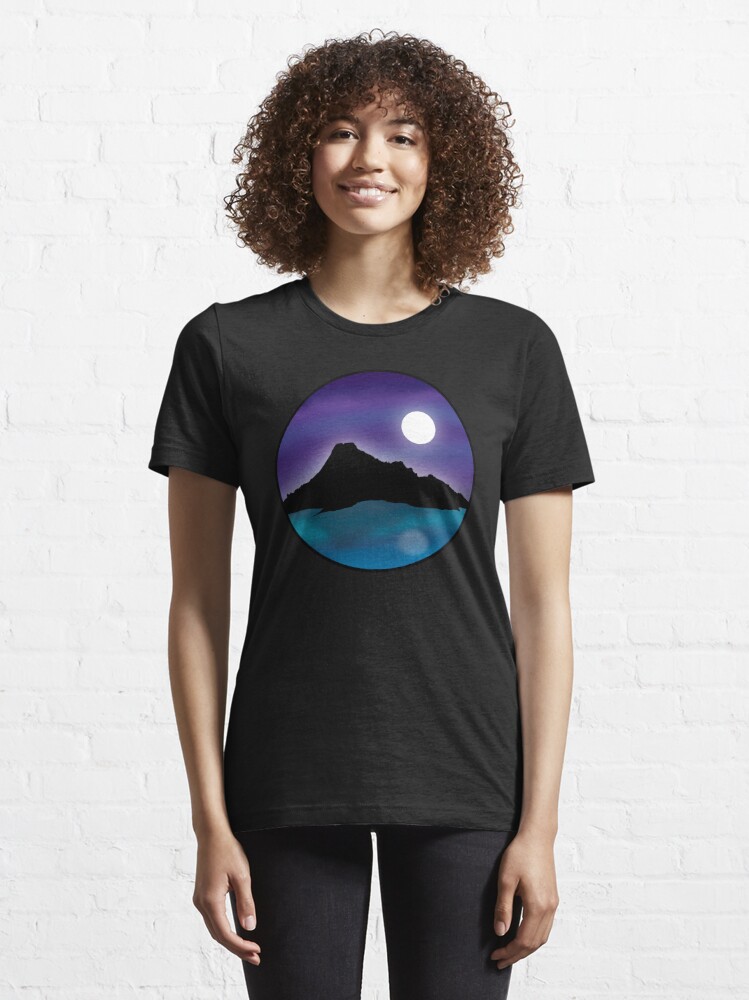A young woman with shoulder-length, very curly dark brown hair and a bright smile stands in front of a white brick wall. She has a light black or olive complexion and is wearing a form-fitting black t-shirt and black leggings or yoga pants. The t-shirt features a prominent circular graphic in the center depicting a black silhouette of a mountainous island. Above the mountains, the hazy sky transitions from a darker to lighter purple, showcasing a bright full moon on the top right. Below the island, the ocean shifts from teal to dark blue, mirroring the moonlight above. The woman, who appears to be African American, has dark eyes and exudes happiness, with her hands resting at her sides.